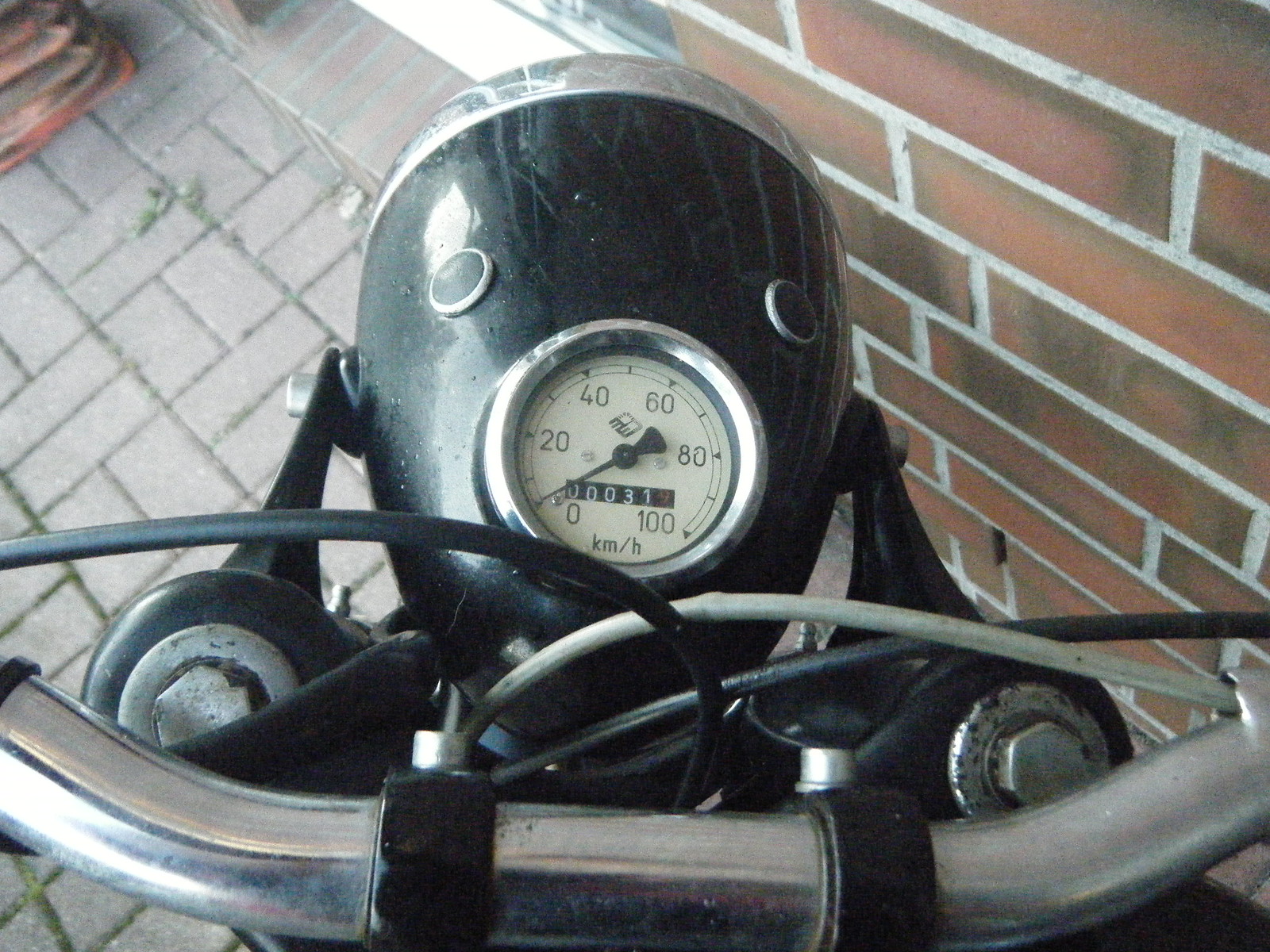This detailed caption encapsulates an amateur photograph of an old, well-worn motorcycle speedometer. The close-up shot makes it difficult to pinpoint specifics, but noticeable features include a speedometer marked in kilometers per hour, going up to 100, and a central odometer, both encased in chrome. The device is mounted on a housing, likely for the headlight, which is black with chrome accents. The handlebars, positioned in proximity to the speedometer, obscure a clear view of the entire vehicle but hint that it is meant to be ridden. The photograph captures a sense of wear and tear, indicative of road use with signs of road dust and minor pings. The setting appears to be a narrow space facing a weathered, medium-red brick wall with a faded red parquet brick floor, suggesting the vehicle is parked very close to the wall, requiring caution to move it without causing scratches. The speedometer's background is white, further emphasizing its vintage state. The photographer’s careful composition indicates they leaned over the handlebars to capture the intricate details of the speedometer and odometer against this meticulously described backdrop.